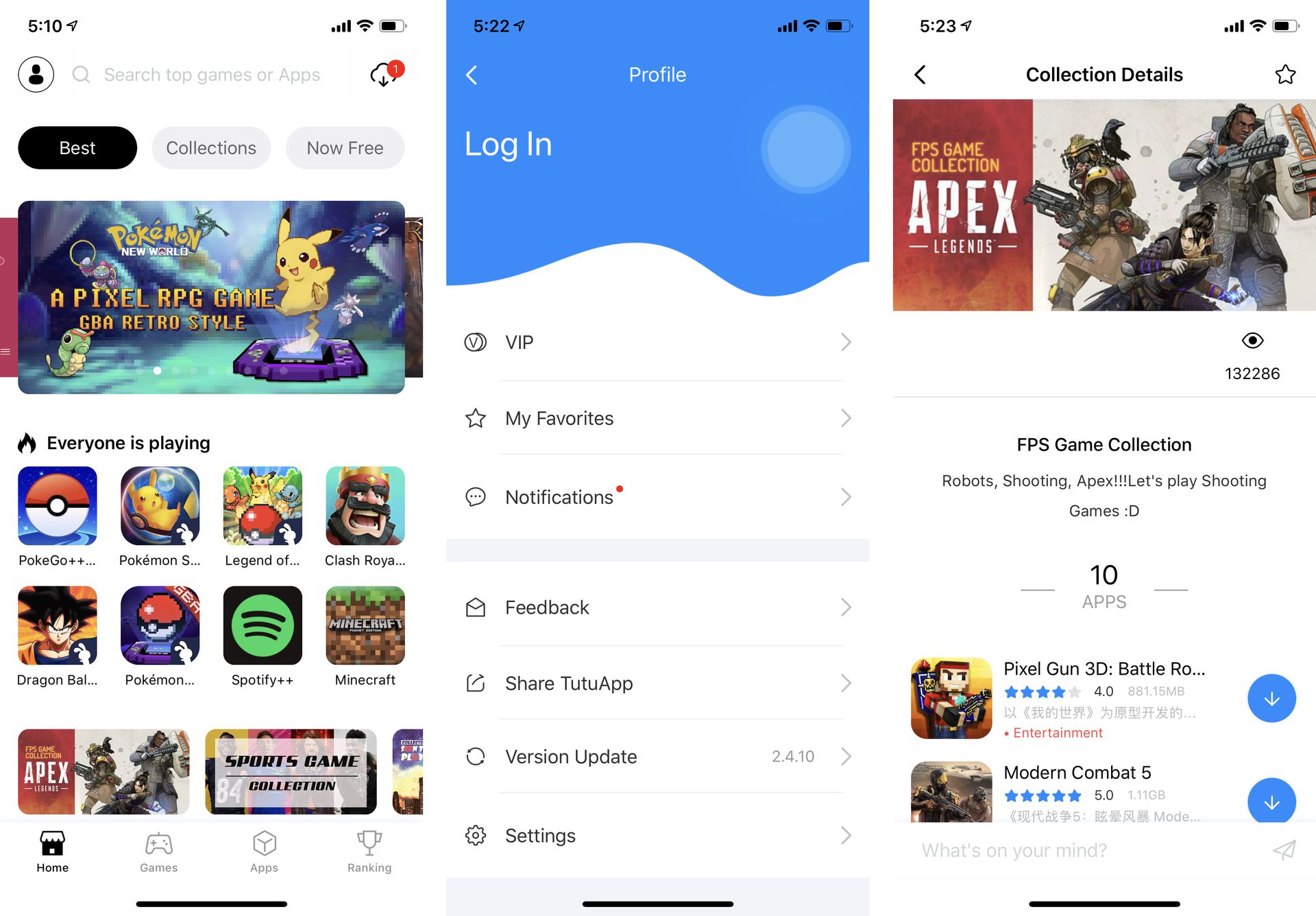The image is a collage of three distinct phone screenshots. The first screenshot, positioned on the far left at the top, displays the number "510" in the upper left corner. The upper right corner contains icons for wireless signal, cellular signal, and battery status. Beneath these icons, a search bar reads "Search Top Games or Apps. Best Collections Now Free." Immediately below, there is an image featuring characters from Pokemon with the text "Pokemon New World, a pixel RPG game, GBA retro style." Below this header, icons for various games, including Pokemon, Dragon Ball Z, and Minecraft, are displayed.

The second screenshot, situated to the right of the first one, shows the number "522" in the top left corner. The top right corner again includes the cellular signal, wireless signal, and battery icons. A list is shown below, which reads: "Profile, Login, VIP, My Favorites, Notifications, Feedback, Share Tutu App, Version Update 2.4.10, Settings."

The final screenshot on the far right depicts the number "523" in the top left corner, with cellular, wireless, and battery status icons in the top right corner. It features a header that reads "Collection Details." Below this, a picture of three anime-styled characters holding weapons is shown with the text "FPS Game Collection Apex Legends." To the left of the picture, it reads "FPS Game Collection Robots Shooting Apex. Let's play shooting games :)".